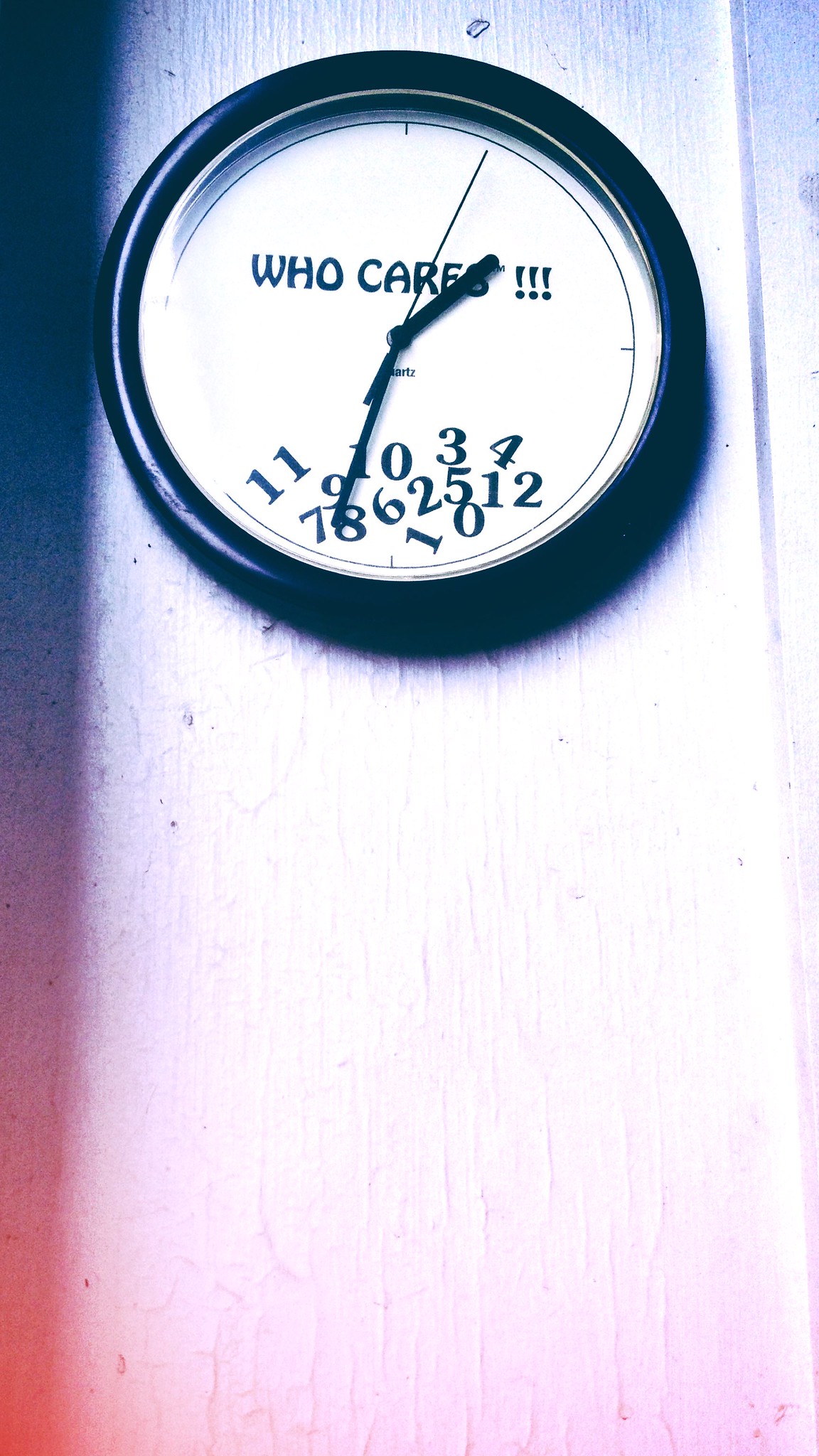The image features a circular clock mounted on a wall, viewed from an upward angle. The clock's design is unconventional, with a black outer frame. The face of the clock prominently displays the phrase "Who cares! ! ! !" in bold letters. The clock hands are positioned such that the hour hand points towards where the 2 o'clock mark would be, while the minute hand aligns roughly with the 7 o'clock position. Instead of being evenly spaced, the numbers 1 through 12 are bunched together at the bottom of the clock face in black font. 

Adorning the wall below the clock is a series of white lights, creating a striking contrast against the timepiece. Starting from the bottom left corner of the image, a gradient of colored lights begins, transitioning seamlessly from pink to purple, then to blue, and finally to a darker blue at the top left corner. These lights add a dynamic and whimsical atmosphere to the composition, highlighting the clock's playful irreverence towards the conventional passage of time.